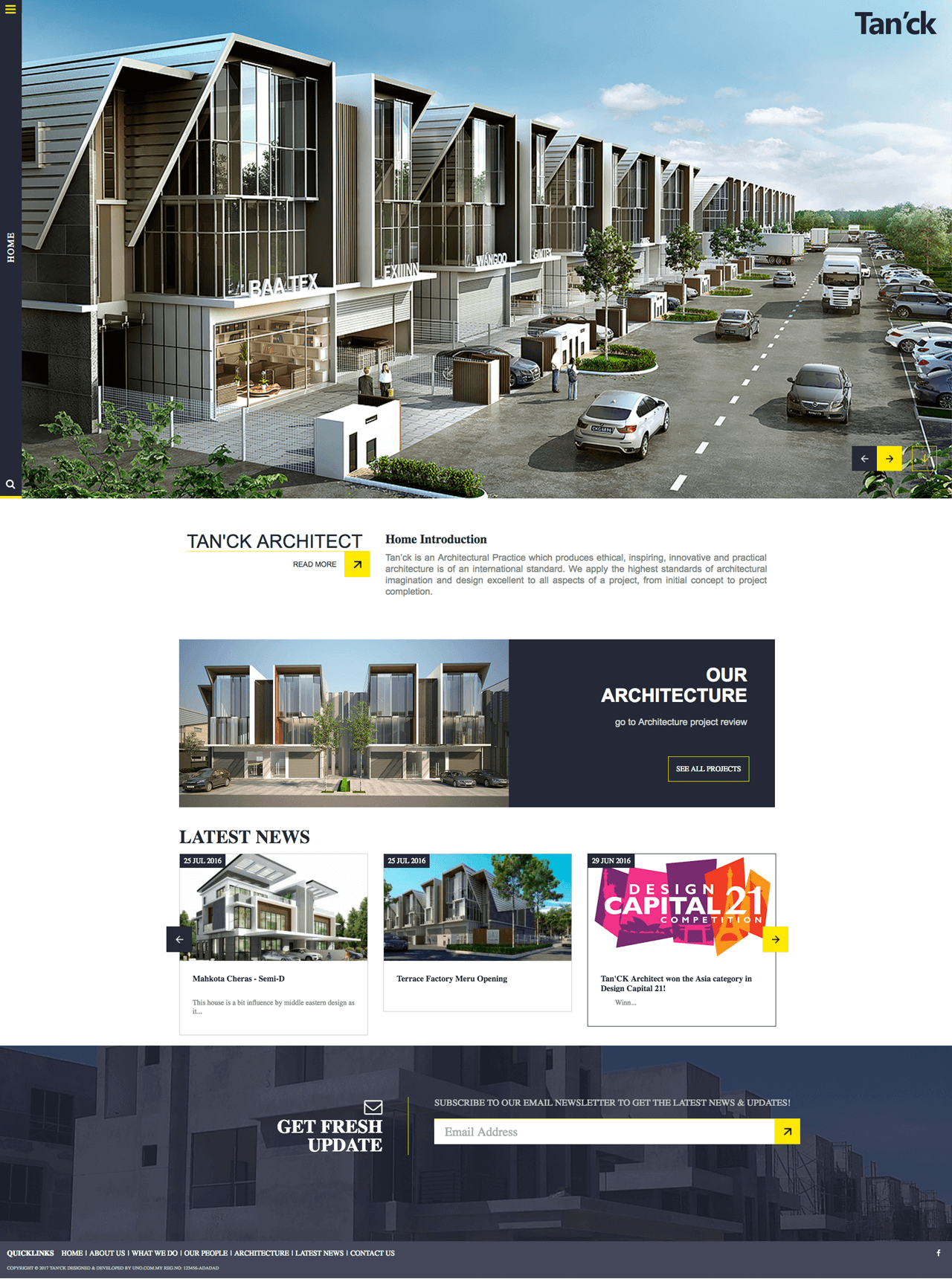The website image displays "TanC K Architect" prominently in the middle, although the text could benefit from being larger for better visibility. Below this heading is a yellow image with links such as "Home" and "Innovation," which could also be more prominent to clearly communicate what the site offers.

At the top of the page, there's an image featuring a series of modern, boxy stores with glass fronts. These stores are captioned with "BEA TEXT" and have signs that suggest the setting is in a foreign country. A driveway runs in front of the stores, dotted with half-donut-shaped cutouts filled with hedges extending to the roadway. Vehicles, including cars and trucks, are seen driving by, and there's a parking lot across from the stores with a covered pull-in area.

Lower on the page, the text "Our Architecture" accompanies a small photo of modern buildings, possibly residential, with garages underneath. The "Latest News" section includes three pictures, two of which are of buildings, and one titled "Design Capital 21," featuring a vibrant mix of purple, orange, yellow, and pink colors. At the bottom, a "Get Fresh Update" section invites users to enter their email addresses into a search bar for updates.